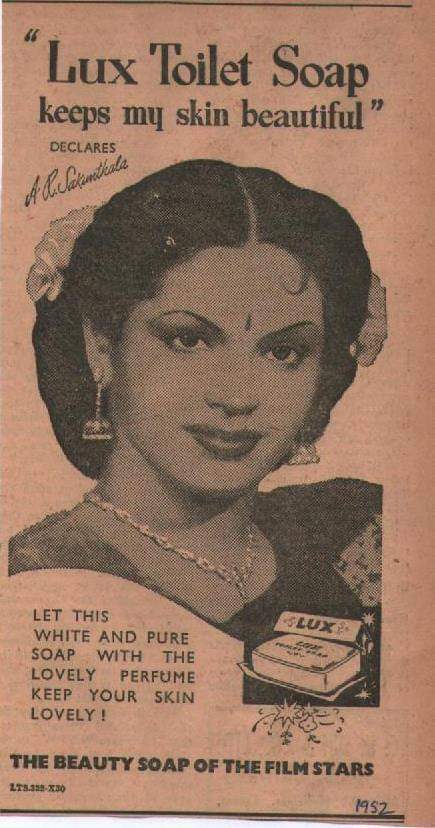This is a photograph of a weathered and faded vintage advertisement for Luxe Toilet Soap, predominantly portrait in orientation. The background displays an aged orangish-pink-peachy hue. At the top, in bold black print and parentheses, the ad declares, "Luxe Toilet Soap keeps my skin beautiful." Below this statement is the cursive signature of an unidentified lady. Central to the image is a bust of a young woman, likely of Indian descent, adorned with flowers in her dark, center-parted hair. She is elaborately styled, featuring heavy eye and lip makeup, long dangling earrings, and a necklace. To the right of her image is an illustration of a Luxe soap bar in its box. Adjacent to it, the text reads, "Let this white and pure soap with the lovely perfume keep your skin lovely." At the bottom of the ad, it proclaims, "The Beauty Soap of the Film Stars." In the lower right-hand corner, a handwritten note in blue ink marks the date as 1952.